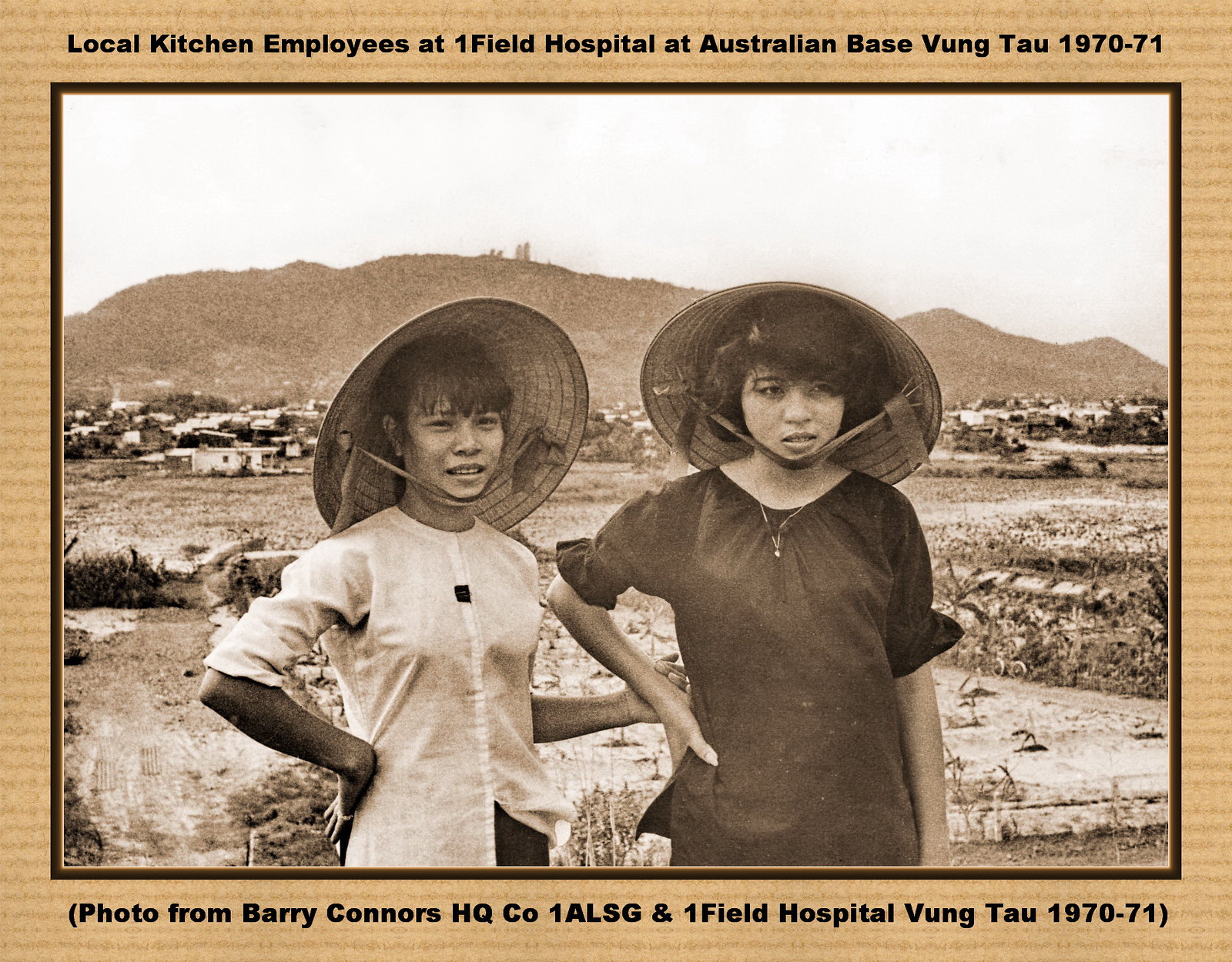This historical black and white photograph, taken between 1970-71, captures two young women believed to be local kitchen employees at the Onefield Hospital within the Australian base in Vung Tau. Both women, possibly in their twenties, stand at the forefront of the image, each donning traditional bonnets. The woman on the left wears a white shirt and appears to be smiling lightly, her hand placed confidently on her hip. Her companion on the right, adorned in a dark shirt and a necklace, exhibits a more serious expression with a similar stance, hands on hips. The background reveals a field leading to some primitive homes or shacks at the base of a hill. This scenic landscape of buildings and mountains, although faint, adds context to the wartime setting. The sepia-toned postcard features a header at the top reading, "Local kitchen employees at Onefield Hospital at Australian base, Vung Tau, 1970-71," and a credit at the bottom, "Photo from Barry Connors, HQ, Co 1 ALSG and Onefield Hospital, Vung Tau, 1970-71."